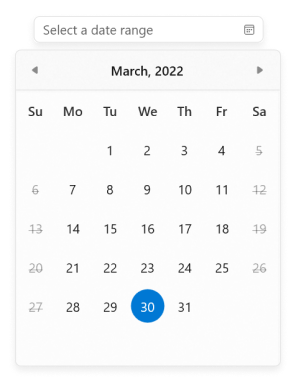This image is a cropped screenshot of a calendar interface, specifically focusing on the "Select Date Range" box. Upon clicking the box, a drop-down calendar appeared. This calendar displays the month of March 2022 at the top, with navigation arrows on either side to scroll through different months. Below the month header, the calendar is presented in a standard format with the days of the week running horizontally from Sunday to Saturday. 

The dates for March 2022 are organized in rows beneath these days, with Wednesday, March 30th prominently highlighted in a blue circle. This highlights that March consists of 31 days, and the final day, March 31st, falls on a Thursday. To the far right within the "Select Date Range" box, there is a calendar icon, indicating that this icon was clicked to reveal the drop-down calendar.